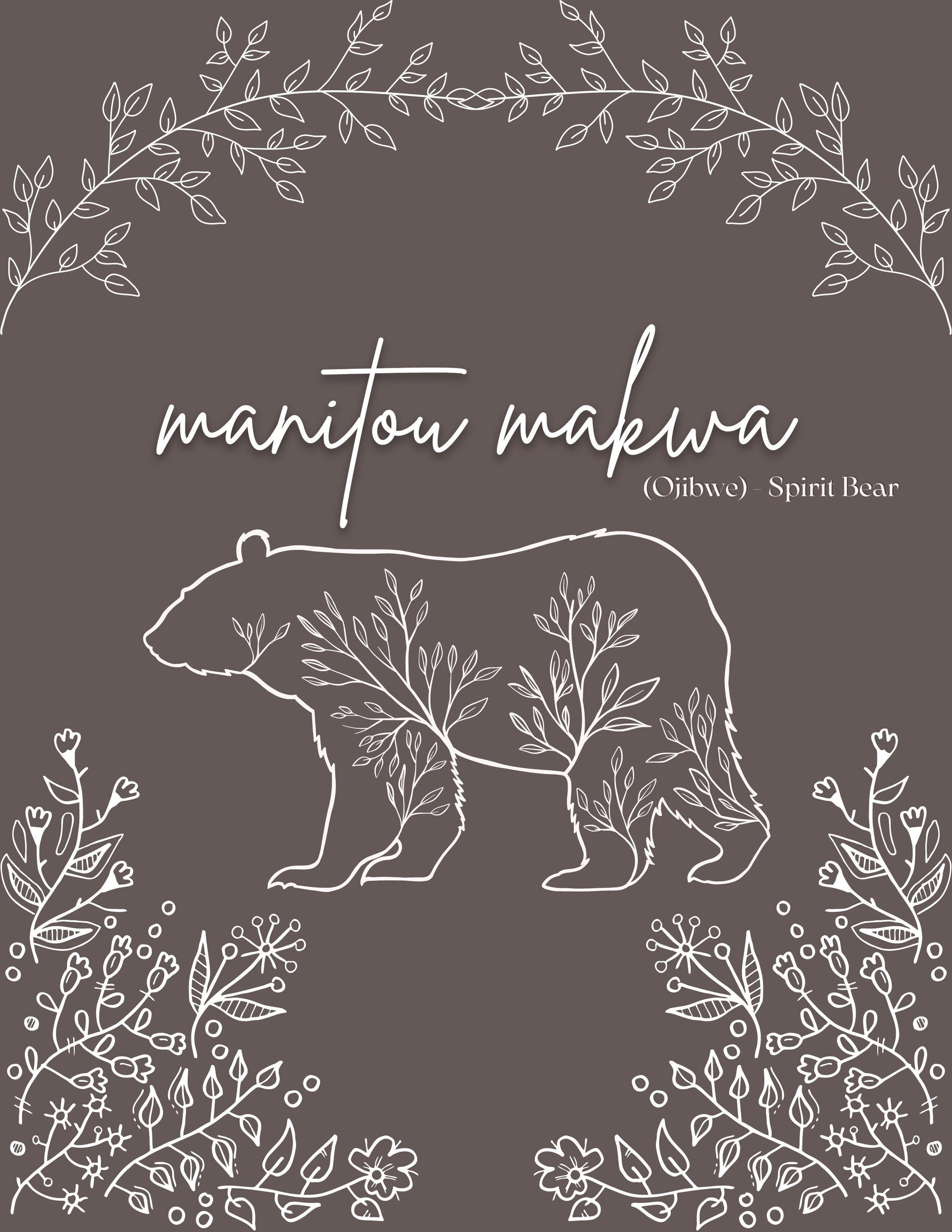The image features a dark gray, almost chalkboard-like background with detailed white illustrations and cursive text. Across the top, a white vine arches from left to right, adorned with long, skinny leaves. Below this vine, cursive text spells out "manitou makwa," followed by the phrase "(Ojibwe spirit bear)" in parentheses. Centrally positioned is the white outline of a bear, filled with artistic representations of tree branches and leaves. The bear's body is intricately interwoven with thin, elongated leaves, creating a forest-like texture. Additional vines with leaves frame the poster, and each bottom corner highlights delicate flowers. The entire piece carries a minimalist yet elegant design, emphasizing the cultural and natural elements depicted.